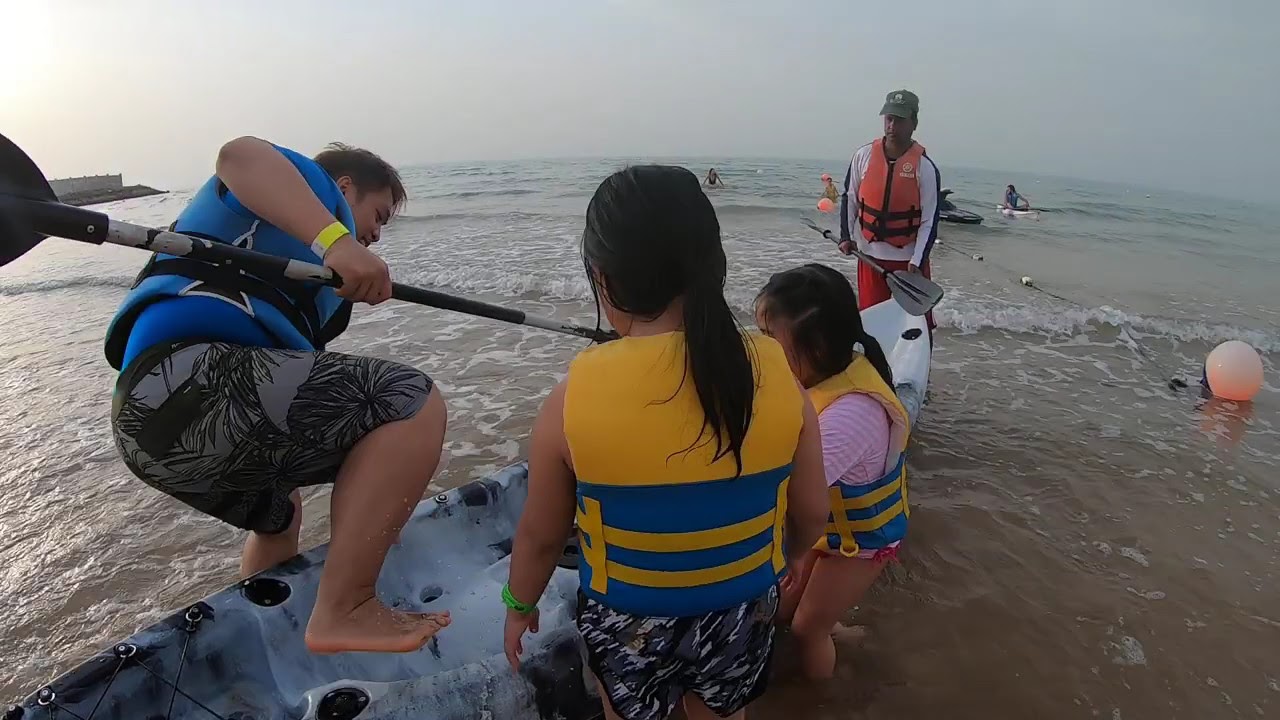This horizontally aligned rectangular photograph captures a detailed scene at the beach, where a man, appearing to be either climbing into or out of a gray and white kayak, is in the shallow, ankle-deep, gray water near the shore. The man, noted for his short brown hair and Caucasian appearance, is wearing a blue life vest and black flowery board shorts with gray patterns. He has an oar in his hand, and a yellow paper bracelet on his right wrist. 

In the foreground, directly in front of the viewer, stands a girl with long dark hair in a ponytail, wearing a yellow and blue life vest over her shorts, showing her back to the camera. Beside her stands another girl, similarly outfitted in a yellow and blue life vest with long dark hair in a ponytail, both seemingly focused on the kayak.

The water is shallow, and beyond the central figures, there's another man, distinguished by his orange life vest, a cap, long-sleeve white shirt, and red trunks. He is holding an oar and appears to supervise the scene or possibly guide the others. 

The background of the image includes additional kayakers playing in the distance, evident with their presence in the sea further out, one with a raft. Additionally, a buoy, described as a pink-colored sphere, is visible on the right side of the image alongside a barrier that seems to demarcate a controlled swimming or boating area. The overall setting is overcast, indicated by the gray hue of both the water and the sky.